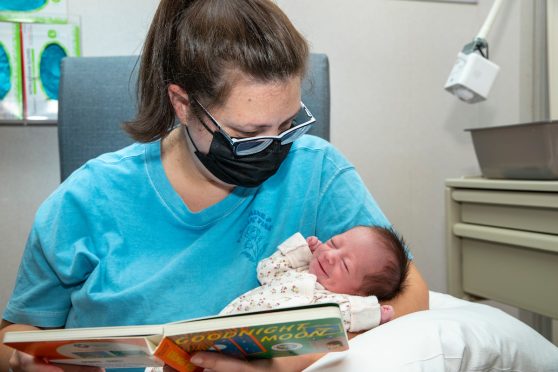In a hospital or medical office setting, a woman, possibly a nurse or mother, is captured in a tender moment reading "Goodnight Moon" to a newborn baby she cradles lovingly in her arms. The woman is seated in a light blue chair and wears a black face mask and glasses with black rims and white inside. Her long brown hair is tied back in a ponytail, and she is dressed in a comfortable, short-sleeved light blue t-shirt. The baby, dressed in a tan long-sleeve outfit with small designs and with short brown hair, appears to be stretching and possibly smiling, with its hands up by its head. The woman's arm, which holds the open book, rests on a white pillow supporting the baby in the crook of her elbow. In the background, there's a white wall adorned with open boxes of gloves on the left-hand side, their blue content peeking through. Drawers are visible on the back right, adding to the clinical atmosphere. Both the woman and the baby seem to share a quiet, joyful connection in this serene snapshot.